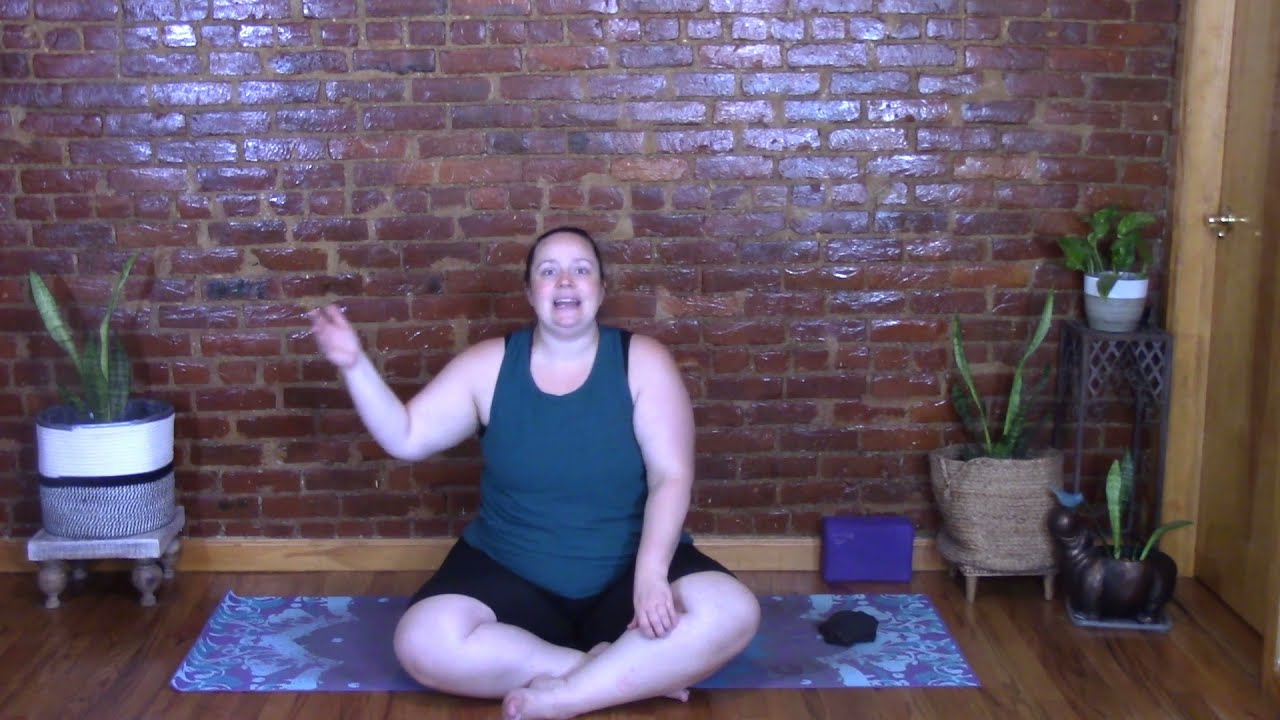The photograph captures a white woman, slightly heavy-set, seated in a cross-legged position on a yoga mat, which features a blue and white pattern, resting on a hardwood floor with vertical brown planks. She is wearing black shorts and a greenish-blue tank top. She has short, dark hair pulled back, and her left arm rests on her leg while her right arm is raised. She faces the camera with her mouth open, suggesting she is recording a video. Behind her is a reddish-brown brick wall accented with light wood molding at the base. To her right, there is a light brown wooden door with a gold doorknob. Surrounding her are various plants in different colored and shaped pots, with some plants positioned on small four-legged platforms. The room is illuminated such that light highlights two spots on the brick wall.